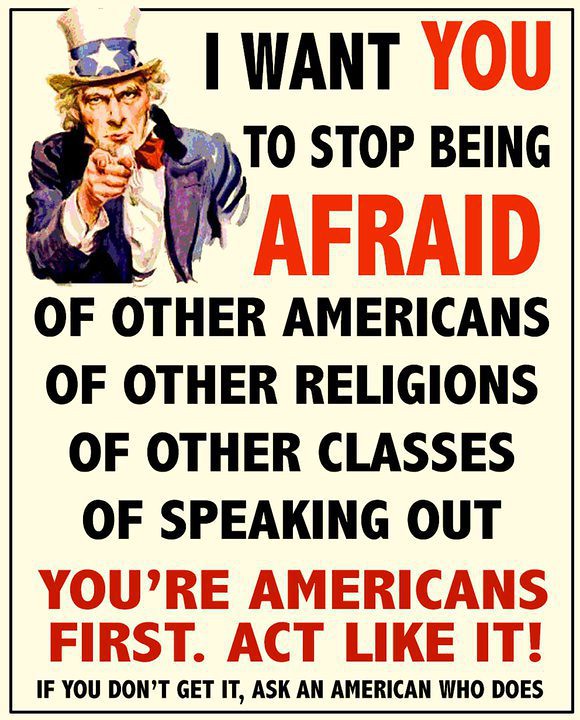The image features a vintage-style illustration of Uncle Sam positioned in the top left corner, pointing directly at the viewer. Uncle Sam is depicted wearing his iconic white top hat, which has a blue band adorned with white stars in the front. He sports a blue jacket, a white long-sleeved shirt, and a reddish tie. His distinct facial features include a long gray goatee and some curly hair peeking out from under his hat.

The image is outlined in black and includes a significant amount of text in both black and red. The red text emphasizes important words: "you," "afraid," and the phrase "you're Americans first, act like it." The complete message reads: "I want you to stop being afraid of other Americans, of other religions, of other classes, of speaking out. You're Americans first, act like it! If you don't get it, ask an American who does." The sign delivers a positive and motivational call to unity and courage, encouraging viewers to overcome their fears of different groups and to embrace their shared identity as Americans.